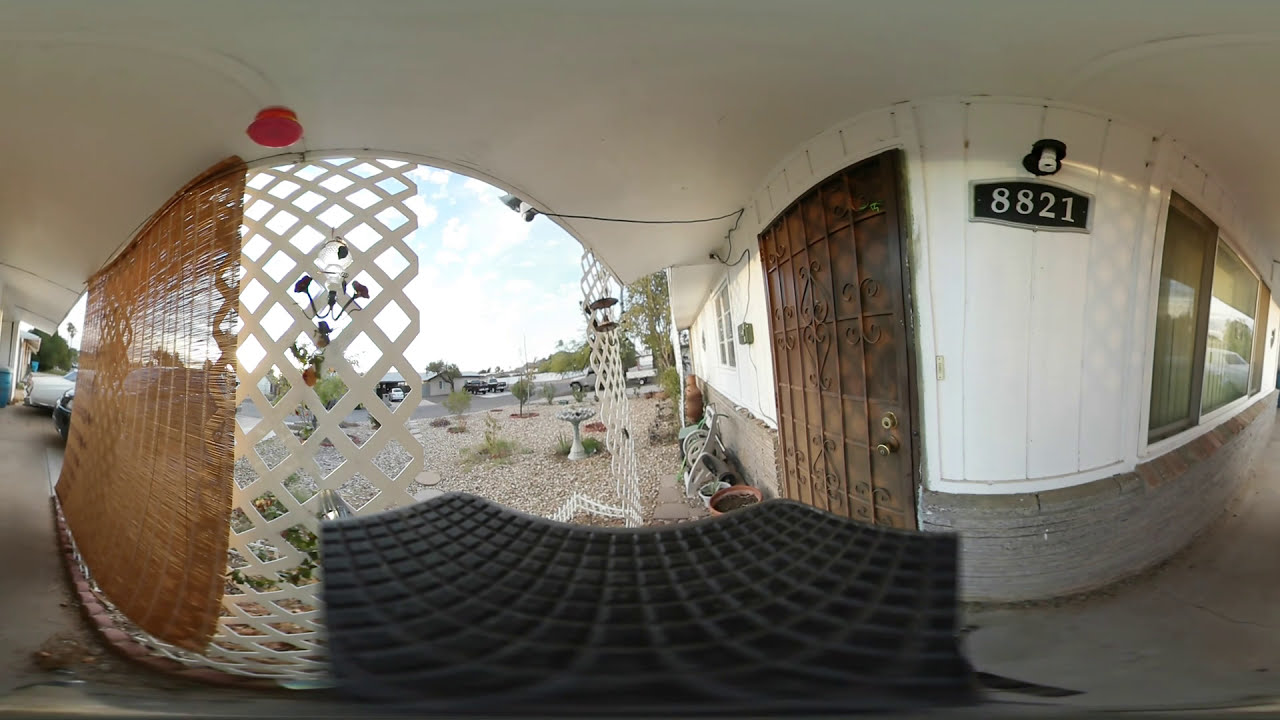The image captures the front entrance of a home in a desert-like terrain, likely in the southwestern United States, taken with a fisheye lens for a panoramic effect. Dominating the scene is a heavy brown door positioned centrally on a white house, flanked by a white doorbell to its right and the house number "8821" displayed on a black sign with grey or white font to its left. Above the sign, a light bulb illuminates the entryway.

The porch area is covered and features a welcome mat directly in front of the door. To the left, a bamboo shade hangs over a trellis-type latticework providing shade. Below the latticework, a sidewalk extends, with cars visible further down. To the right of the door, a black grate can be seen along with a water hose and some potted plants, emphasizing the arid environment devoid of grass, substituted with rocky, river wash landscaping.

The image also captures additional latticework, the gravel yard, and parts of the driveway and roadway area outside the home, blending into the broader desert landscape of the estate.